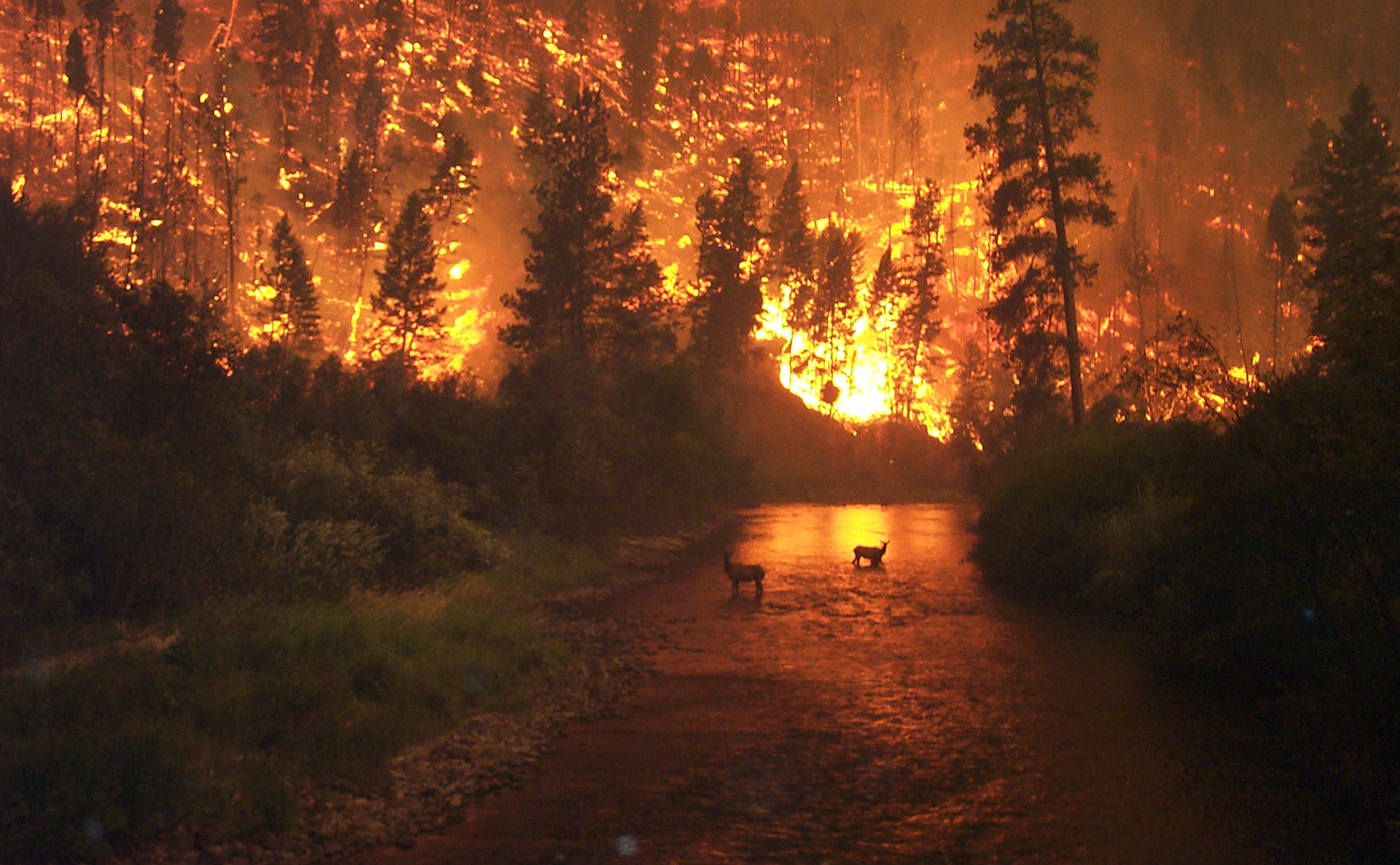The image depicts a harrowing scene of a forest fire, reminiscent of the devastating California wildfires from recent years. It is nighttime, as evidenced by the absence of sunlight, with the primary sources of light being the intense orange and yellow flames that dominate the landscape. The fire, consuming the scenery, spans across the left and right sides, with trees and bushes engulfed in the inferno, suggesting the blaze is spreading across hilly or mountainous terrain.

In the foreground and middle section of the image, there appears to be a narrow strip of land untouched by the flames, perhaps a walkway or clearing. Within this untouched area, two small animals stand outlined against the fiery backdrop. These creatures, possibly young deer or dogs, add a poignant touch to the chaotic and destructive atmosphere, highlighting the impact of the fire on wildlife. The smoke and dark-colored fog hang heavily in the air, further emphasizing the severity of the wildfire and the dramatic, oppressive nature of the scene.